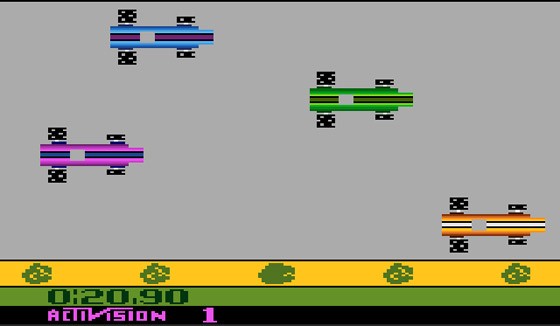This image captures a still from a classic video game by Activision. A black bar at the bottom of the screen displays the text "Activision 1." Directly above it, the number "20.90" is prominently shown. The image features a yellow bar with small green images, likely indicating some form of game information or status. Dominating the scene is a gray roadway on which four cars are positioned. The top car is blue with a purple stripe, followed by a green car with a darker green stripe. Below them is a light purple car adorned with a blue stripe, and finally, a yellow car with a white stripe. Each car's tires are depicted as blocky shapes with white lines, emphasizing the retro, pixelated art style of this old-school video game.